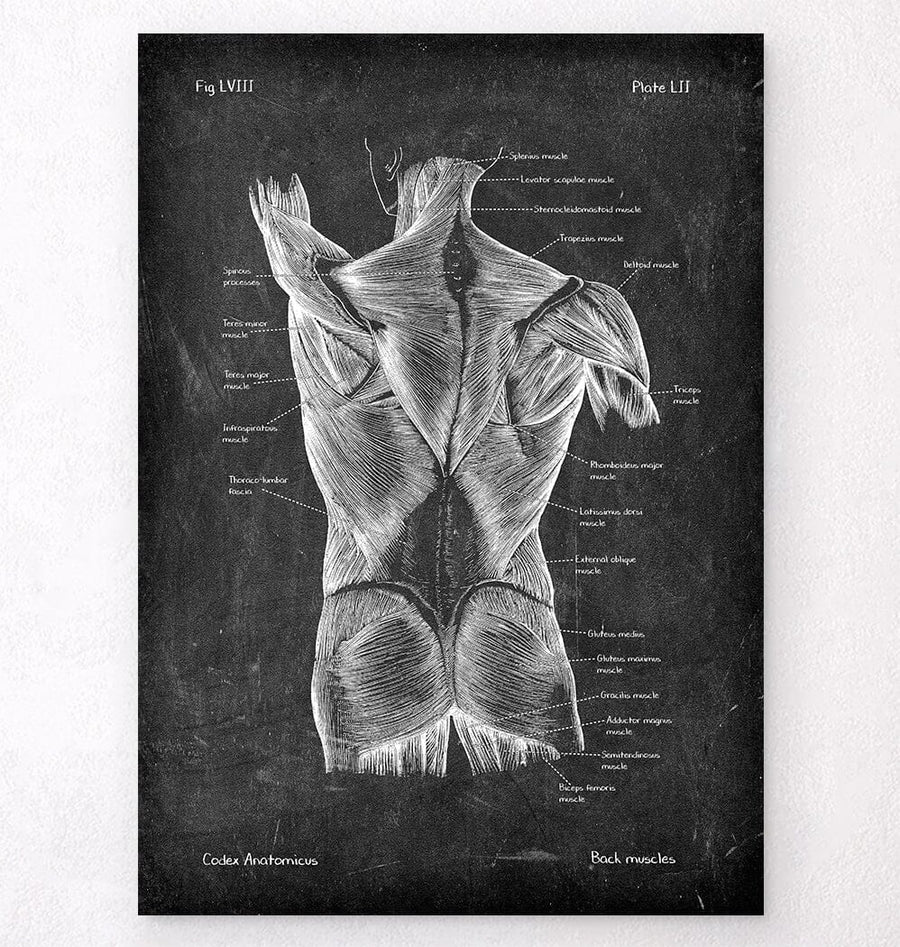The image features a scientific diagram set against a black background, designed to replicate the appearance and texture of a chalkboard. At the top left corner, in white Roman numerals, it reads "FIG LVIII" (58) and on the top right, "PLATE LII" (52). The illustration details the anatomy of a human figure from behind, meticulously showcasing the various muscles through distinct white striations and linings. Each muscle group is labeled with white text, accompanied by lines pointing to specific areas, although the text is somewhat small and hard to read clearly. The diagram spans from the base of the skull through the back, upper arms, chest, down to the buttocks and upper thighs. At the bottom of the image, in white text, "CODEX ANATOMICUS" is inscribed on the left side and "BACK MUSCLES" on the right, further emphasizing the detailed anatomical focus.